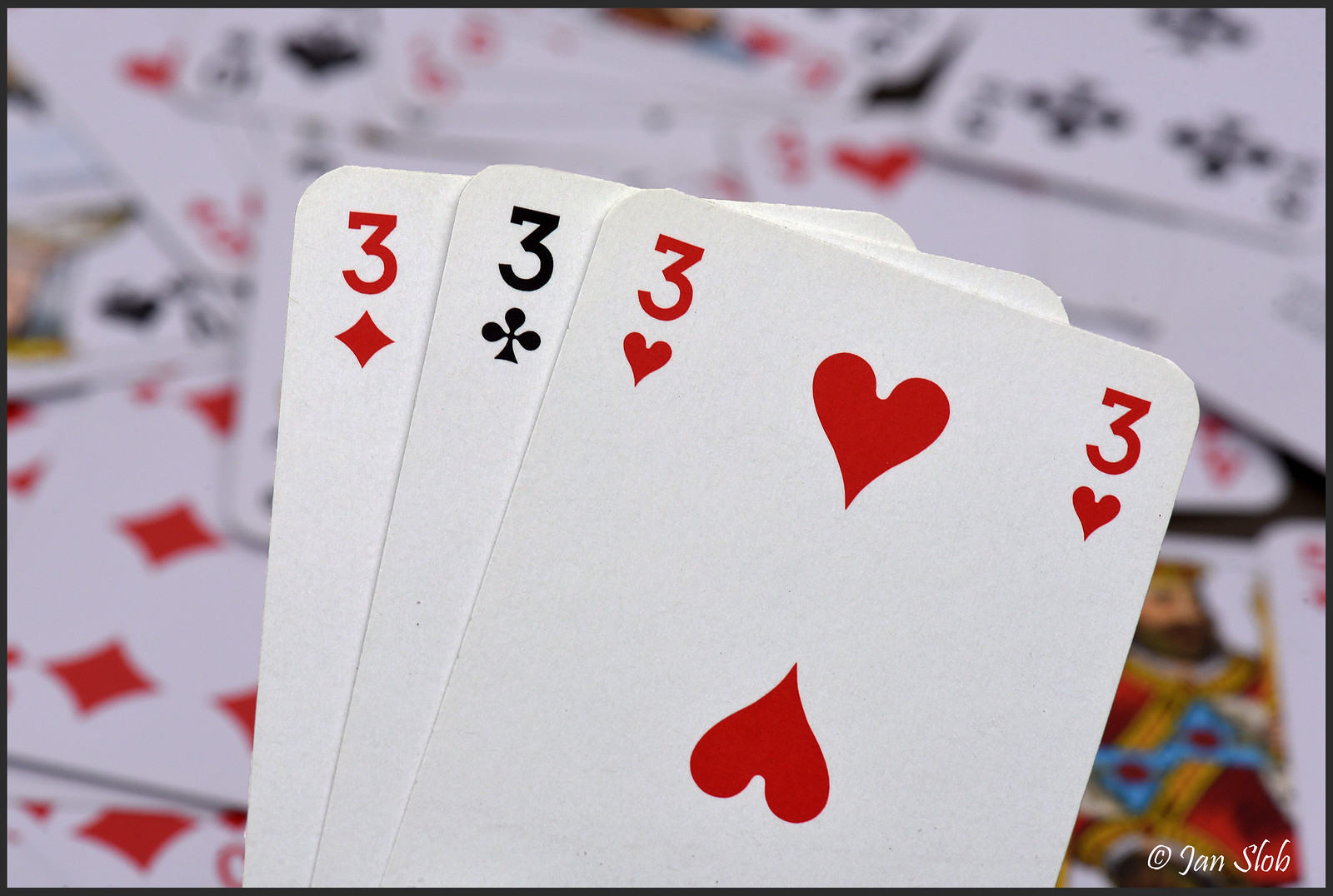A detailed image depicts a scene of intense card-playing. Encased in a thin black border, the centerpiece of the photo features a vertical arrangement of three prominent cards, rising from the bottom about two-thirds of the way up. The card on the left is partially hidden, only revealing the three of diamonds. Stacked above it is the three of clubs, and at the pinnacle, slightly to the right, lies the three of hearts. The three of hearts card displays the number and heart symbols in the top left and right corners, with an upright heart in the middle, slightly to the right, and an upside-down heart below it, angled to the left.

In the bottom right corner, the name "Jan Slob" is inscribed in white lettering. The background, though blurry, is a chaotic spread of various scattered cards. Notably, in the bottom left corner, partially concealed behind the foreground cards, is what appears to be a full display of diamonds. Above this, the queen of spades and another card, likely a heart, are visible. The top section of the image shows hints of other cards, including a discernible club in the top right corner, a king card whose suit is indeterminate, and a card with red markings near the right edge of the frame—that card's suit remains unclear. The blend of distinct and indistinct elements captures the tumultuous essence of a card game in progress.